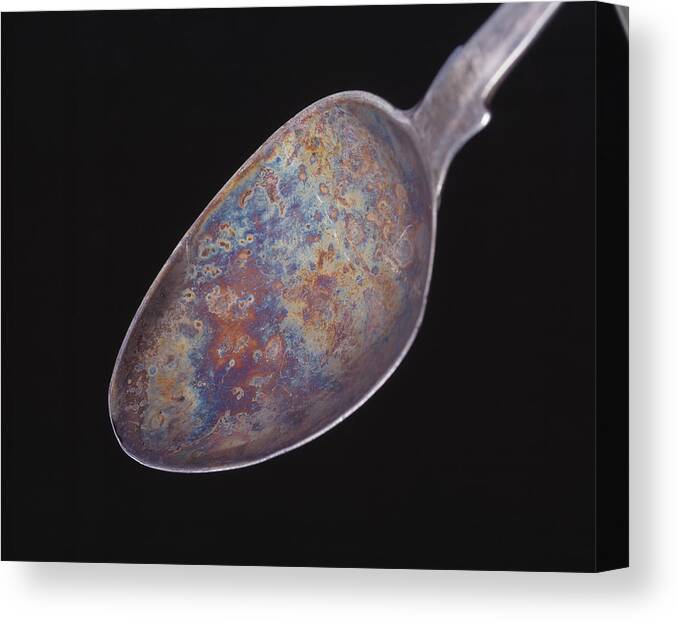This is an up-close photograph of a very old, extremely rusty silver spoon set against a completely black background. The spoon, slightly tilted with the right side closer to the camera, is positioned at the center of the image. The oval-shaped bowl of the spoon, which dominates the center of the frame, is heavily rusted and displays a palette of colors including blue, black, green, brown, and yellow. The handle extends from the top right corner, descending diagonally towards the bottom left corner. Despite the corrosion, there are still small patches of the original silver visible, particularly in the top right corner. The background's stark blackness emphasizes the intricate, multicolored rust patterns and the spoon's worn, bent appearance, suggesting extensive use over time.